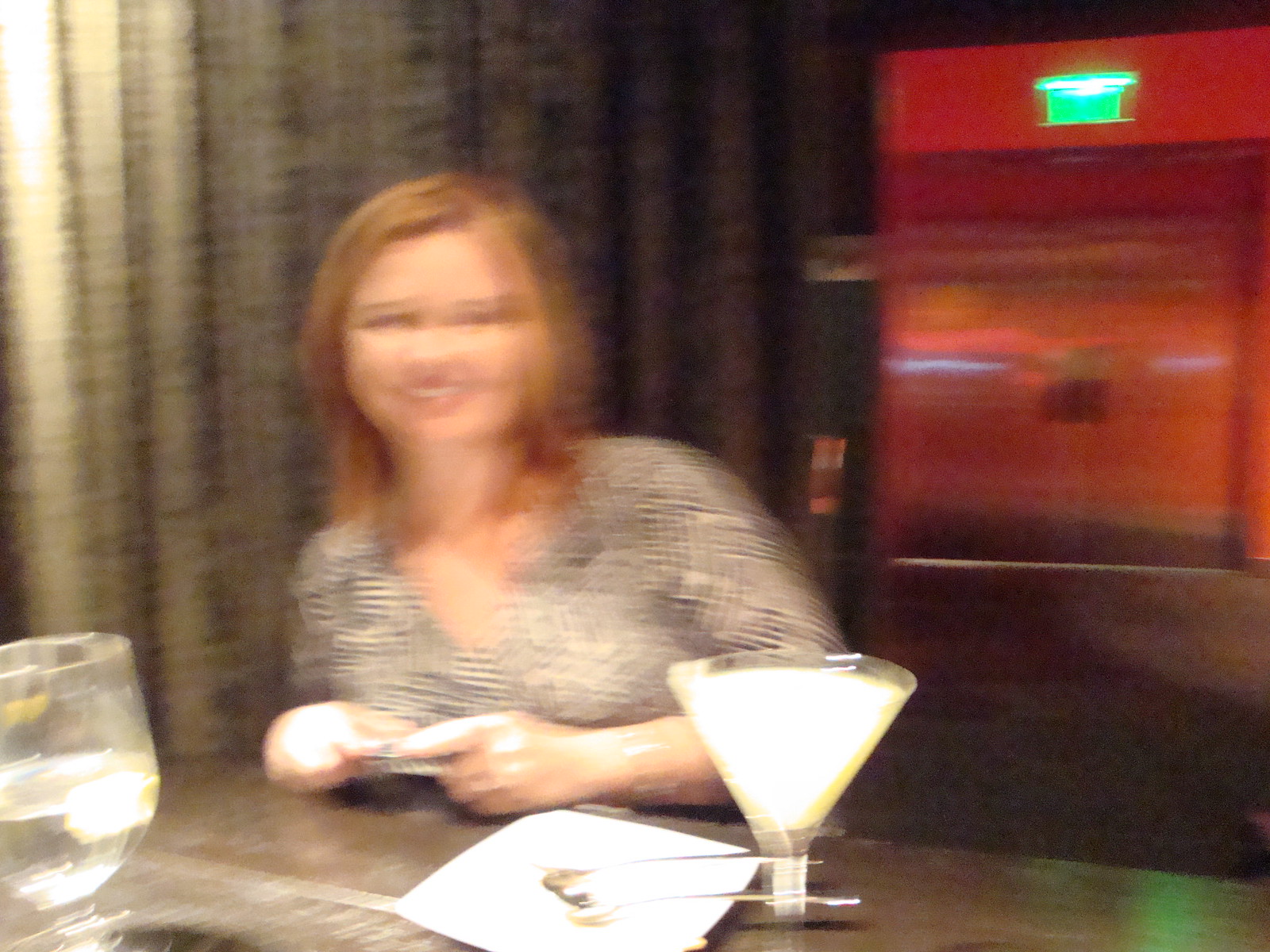The image is a blurred depiction of a Caucasian woman with light brown to reddish brown, shoulder-length hair, smiling warmly at the camera. She is dressed in a black and white shirt with a crosshatch pattern and is seated at a brown table or bar. Both of her hands rest on the table in front of her. To her lower right sits a martini glass containing a whitish-golden liquid, likely a vodka drink, while to her lower left, a goblet with clear liquid, possibly water, can be seen. Adjacent to the martini glass, slightly to the left, there is a square white plate, which might have sushi on it. The background features a tan curtain and a pair of doors, with a green exit sign overhead, hinting that the scene is set in a bar area possibly leading to a hallway with brown flooring.